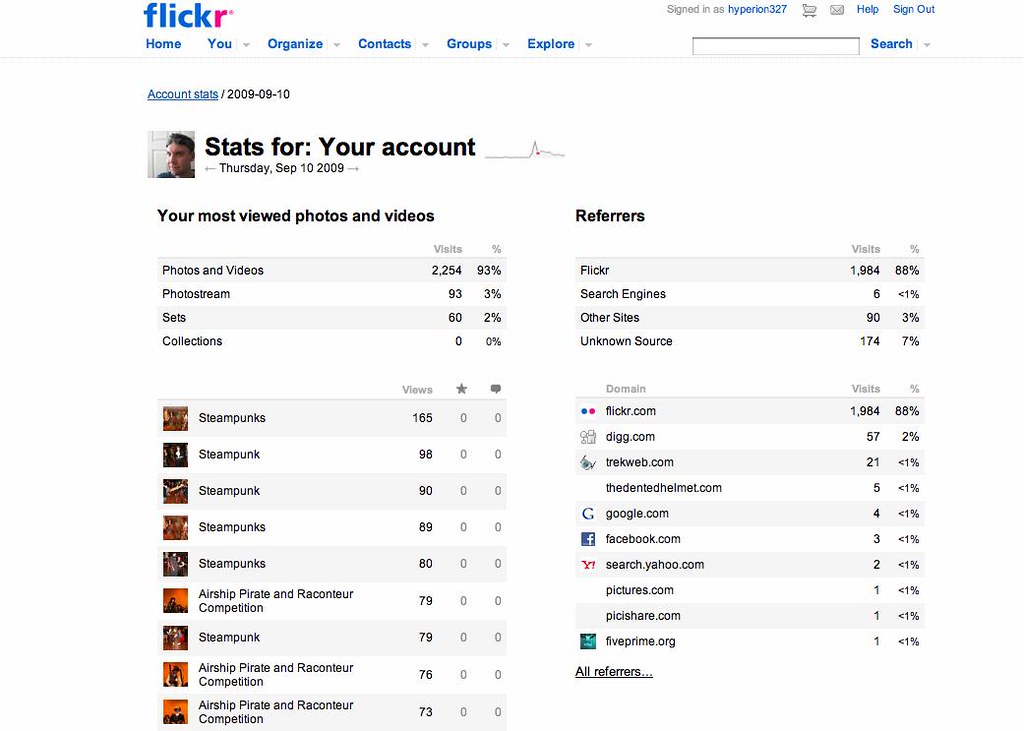The rectangular website screenshot features various account statistics displayed on a predominantly gray or white background. In the top-left corner, blue text reads "Flickr" and is followed by additional blue text links: "Home," "You," "Organize," "Contacts," "Groups," and "Explore." 

Beneath these navigation links, the main section titled "Stats for Your Account" is introduced with an accompanying photograph of a man. Directly below, there's a date marker reading "Thursday, September 10, 2009."

The section continues with "Your Most Viewed Photos and Videos," organized into two columns and two rows. The left column lists:
- **Photos and Videos:** 2,254 visits (93%)
- **Photo Stream:** 93 visits (3%)
- **Sets:** 60 visits (2%)
- **Collections:** 0 visits (0%)

To the right, the second column highlights:
- **Flickr:** 1,984 visits.